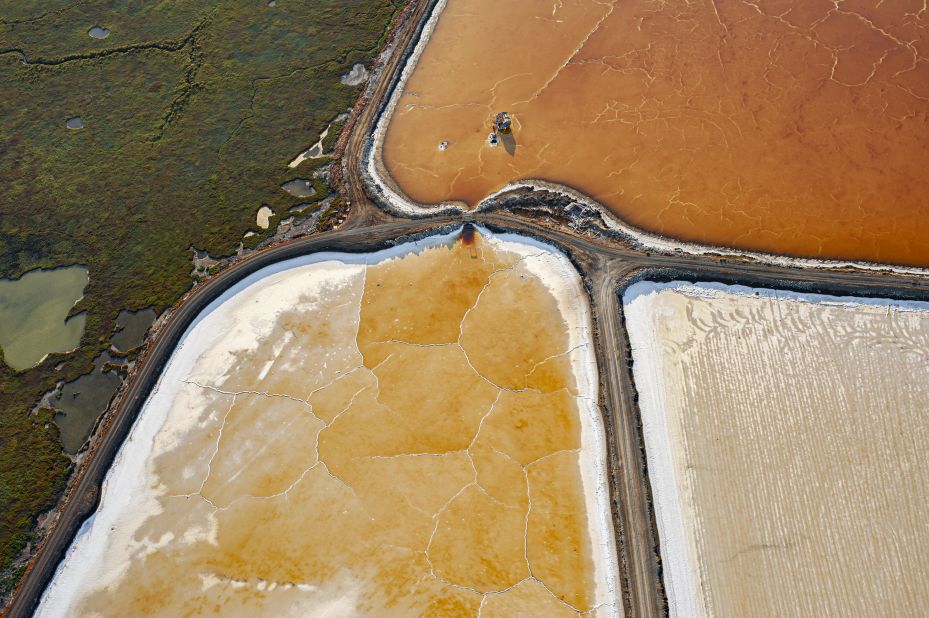This aerial view captures a captivating landscape divided into distinct sections. In the top right quadrant, there is a pond with an orange and brown cracked surface, surrounded by a white border. The lower left quadrant features a pond the color of baked bread, with prominent white edges that expand outward. Adjacent to this, in the lower right quadrant, is a pond resembling white frosting with a light beige hue and a similar white border. A curved road divides these ponds, weaving from the bottom left towards the center and branching off towards multiple intersections. The upper left quadrant reveals green wetlands with small ponds scattered throughout and tiny houses lining the periphery of the fields. The vivid contrasting colors and intricate details present a mesmerizing patchwork of natural and man-made elements.